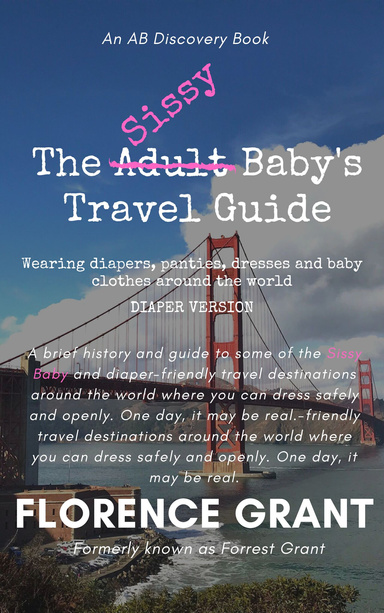The image depicts the cover of a travel guidebook titled "The Sissy Baby's Travel Guide." The background features a wide shot of the Golden Gate Bridge stretching across the San Francisco Bay on a partly cloudy day, with white puffy clouds against a blue sky. In the foreground, an AB Discovery book label is visible in a small white font. The main title, "The Adult Baby's Travel Guide," is prominently displayed, with the word "Adult" crossed out in pink and replaced with "Sissy" in the same pink font. Below the title, a subtitle reads: "Wearing diapers, panties, dresses, and baby clothes around the world, diaper version," in white text. A paragraph of white and pink text elaborates on sissy baby and diaper-friendly travel destinations around the world where people can dress safely and openly. At the bottom, the author's name, Florence Grant, is written in large white letters, followed by "Formerly known as Forrest Grant" in a smaller font. The scene also includes the bay's water with some foam and a brick building near the bridge, adding to the San Francisco locale's charm.